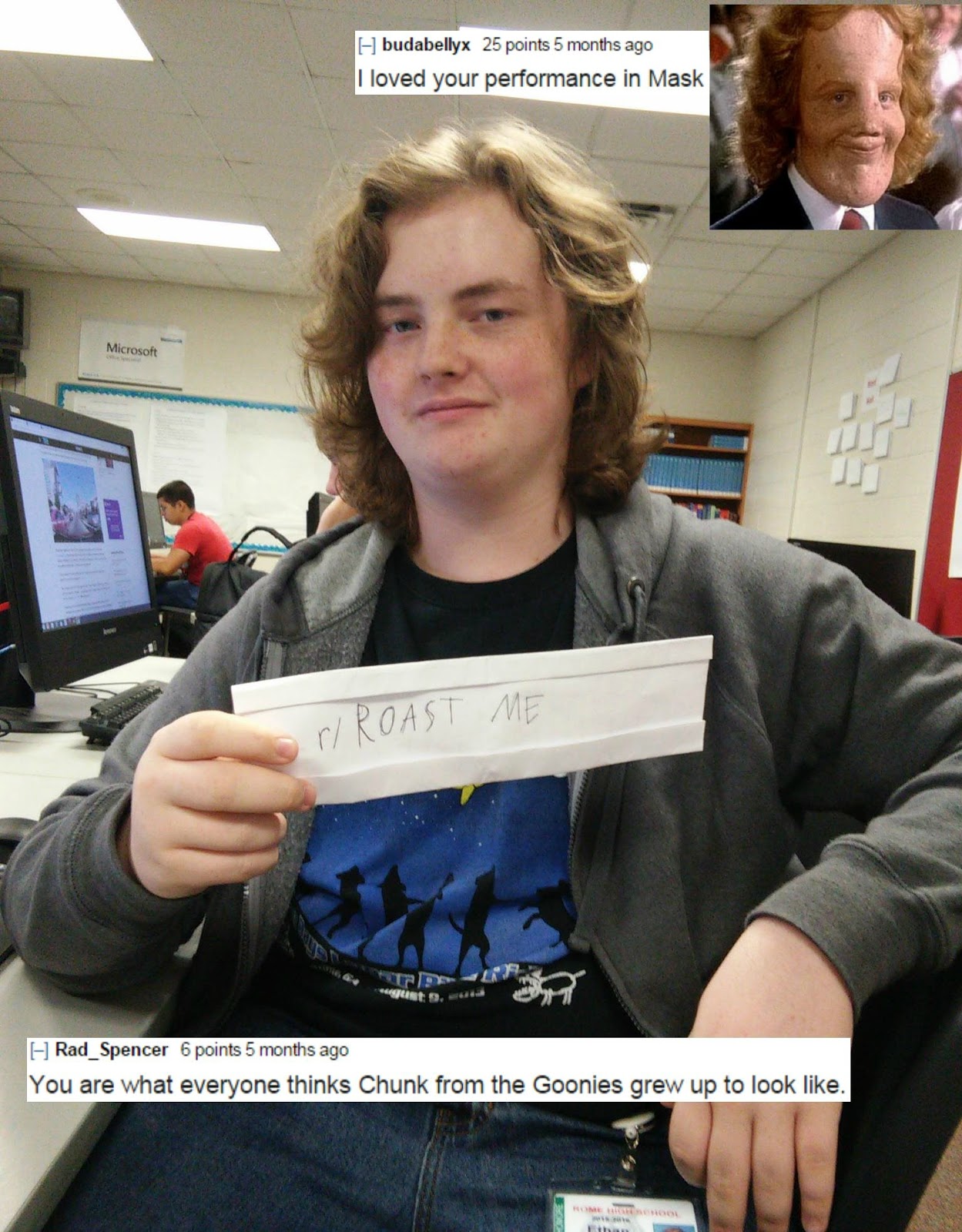The image depicts a young man, likely a high school student aged around 16 to 18, sitting sideways on an office chair in what appears to be a classroom or office setting. He has shoulder-length red hair, a freckled face, and is wearing a graphic tee, hoodie, and jeans. Holding a handwritten sign that reads "r/roastme," he invites insults typical of the subreddit Roast Me. Beside him is a computer, and another student is visible working in the background. The image includes a pasted Reddit comment by Rad Spencer with six points from five months ago, reading, "You are what everyone thinks Chunk from the Goonies grew up to look like." In the top right corner, there's another Reddit post by Bud Balix with 25 points from five months ago that reads, "I loved your performance in Mask," accompanied by a picture of a character from the movie *Mask*, which shares a similar hairstyle and hair color to the student in the photo, enhancing the roasting resemblance.